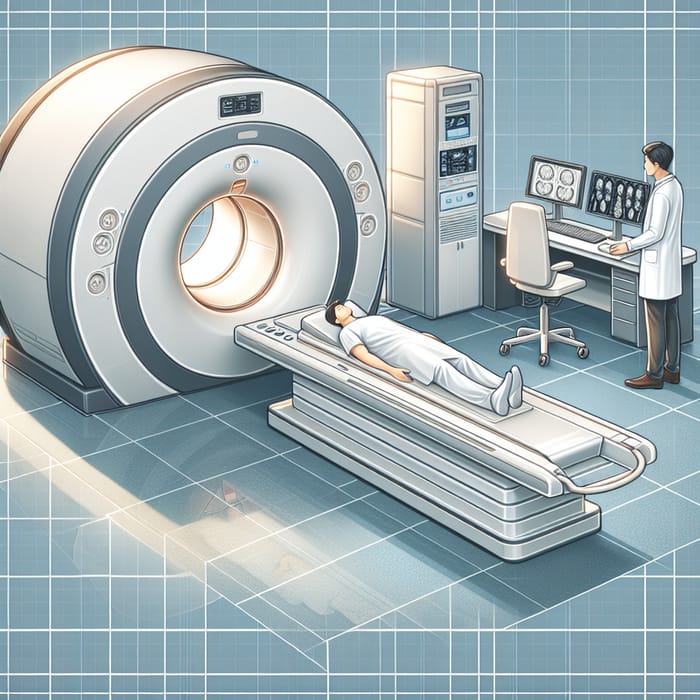This is a detailed color illustration of a medical room featuring an MRI imaging scene. At the center of the image lies the patient, dressed in white clothing and socks, with brownish-black hair, resting his head on a pillow, positioned on the sliding table of a large, cylindrical MRI machine. The MRI machine, primarily white with gray sections, resembles a deep, tire-shaped structure. To the right of the patient stands a doctor, distinguished by a white lab coat and gray pants, who is strategically placed at a desk. The desk hosts multiple computer displays, suggestive of imaging data from the MRI scan. The doctor appears to be operating a computer mouse, likely reviewing the scan results, as various images are visible on the screens. Adjacent to the desk is a white office chair, and nearby is a large, gray and white cabinet filled with data modules and control interfaces. The entire room is accented by a light blue floor adorned with white lines, reiterating the clinical setting.